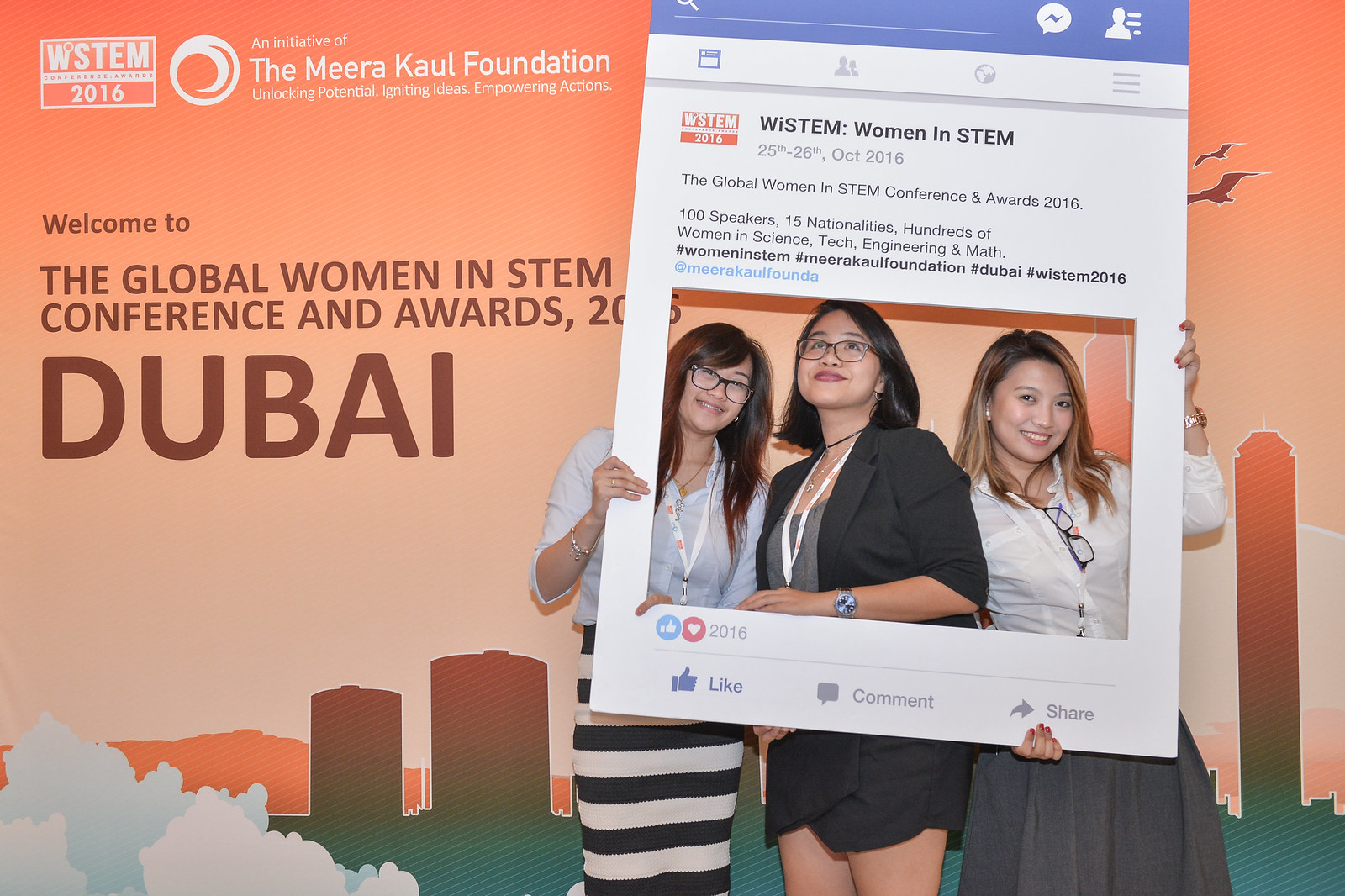In this image, three young Asian women stand in front of a prominently displayed banner for the Meera Kaur Foundation at the Global Women in STEM Conference and Awards 2016, held in Dubai. The banner reads, "The Meera Kaur Foundation, Unlocking Potential, Igniting Ideas, Empowering Action, WSTEM Conference Awards 2016." The women are standing inside a large frame styled to resemble a Facebook post. The frame includes text stating, "WSTEM Women in STEM, 25th - 26th October 2016, The Global Women in STEM Conference and Awards 2016, 100 speakers, 15 nationalities, hundreds of women in science, tech, engineering, and math," along with numerous hashtags including #WomenInSTEM, #MeeraKaurFoundation, and #Dubai.

Dressed in formal attire, two of the women wear white button-up shirts paired with dresses, while the woman in the center sports a business suit. All three wear glasses and exude a youthful, professional demeanor. The orange background behind them reads, "Welcome to the Global Women in STEM Conference and Awards 2016, Dubai." The frame also displays elements typical of a social media post, such as 'likes' and 'loves' icons, highlighted under the year 2016.